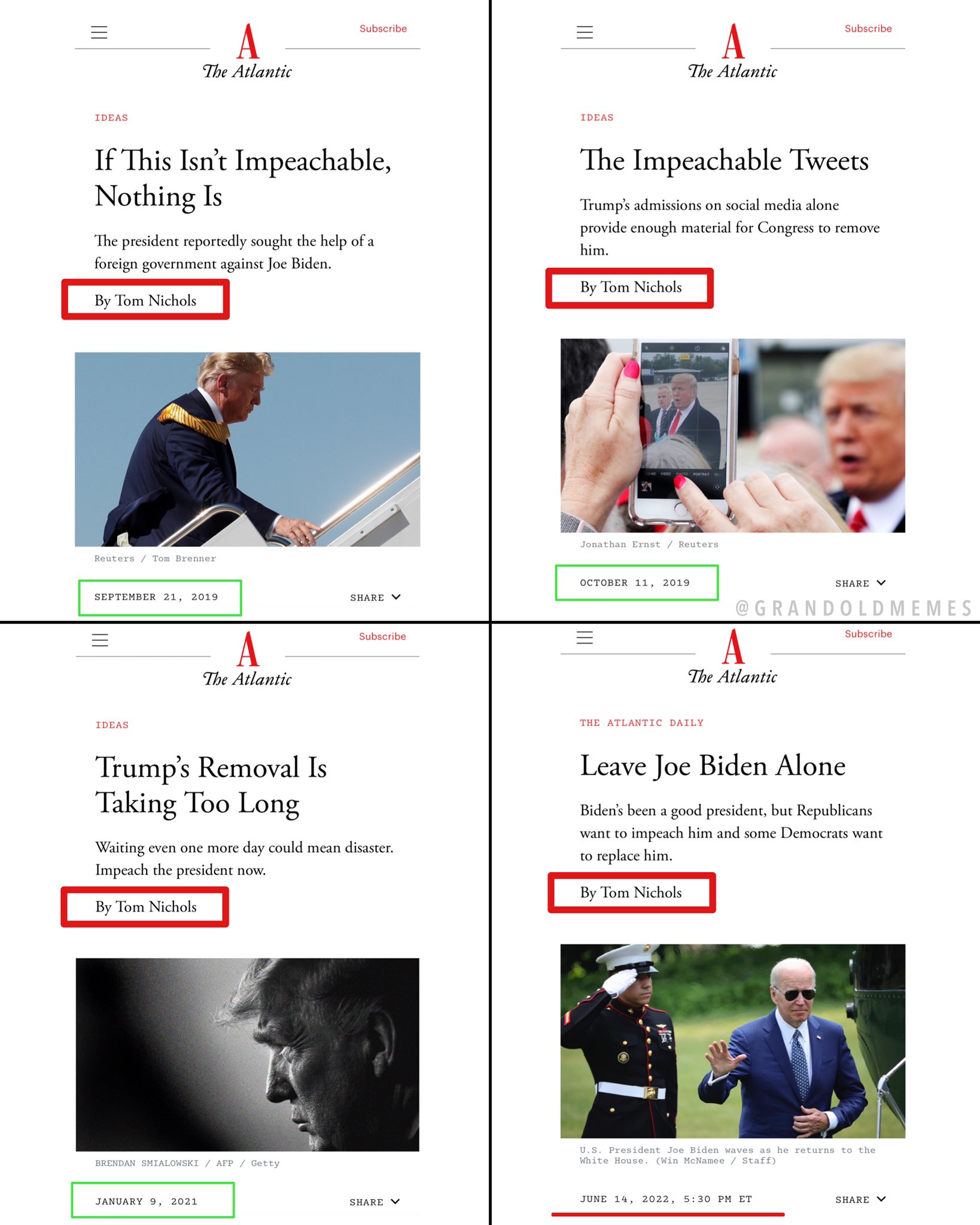The image consists of four distinct graphics, each seemingly sourced from The Atlantic's website, sharing a similar layout and aesthetic.

**Top Left Graphic:**
- **Headline:** "If This Isn't Impeachable, Nothing Is"
- **Subtext:** "The president reportedly sought the help of a foreign government against Joe Biden."
- **Author:** Tom Nichols (highlighted in a red rectangle)
- **Image:** Donald Trump walking up a white staircase towards a plane, set against a blue backdrop.

**Top Right Graphic:**
- **Headline:** "The Impeachable Tweets"
- **Subtext:** "Trump's admissions on social media alone provide enough material for Congress to remove him."
- **Author:** Tom Nichols
- **Image:** A person with pink nail polish holding up a cellphone to photograph Donald Trump, who is visible in the background.

**Bottom Left Graphic:**
- **Headline:** "Trump's Removal is Taking Too Long"
- **Subtext:** "Waiting even one more day could mean disaster. Impeach the president now."
- **Author:** (implied to be Tom Nichols, given the context)

**Bottom Right Graphic:**
- **Headline:** "Leave Joe Biden Alone"
- **Subtext:** "Biden's been a good president, but Republicans want to impeach him, and some Democrats want to replace him."
- **Image:** Joe Biden in a suit, flanked by saluting military personnel.

The overall composition presents a series of critiques and opinions regarding the impeachment processes and political dynamics involving Donald Trump and Joe Biden.